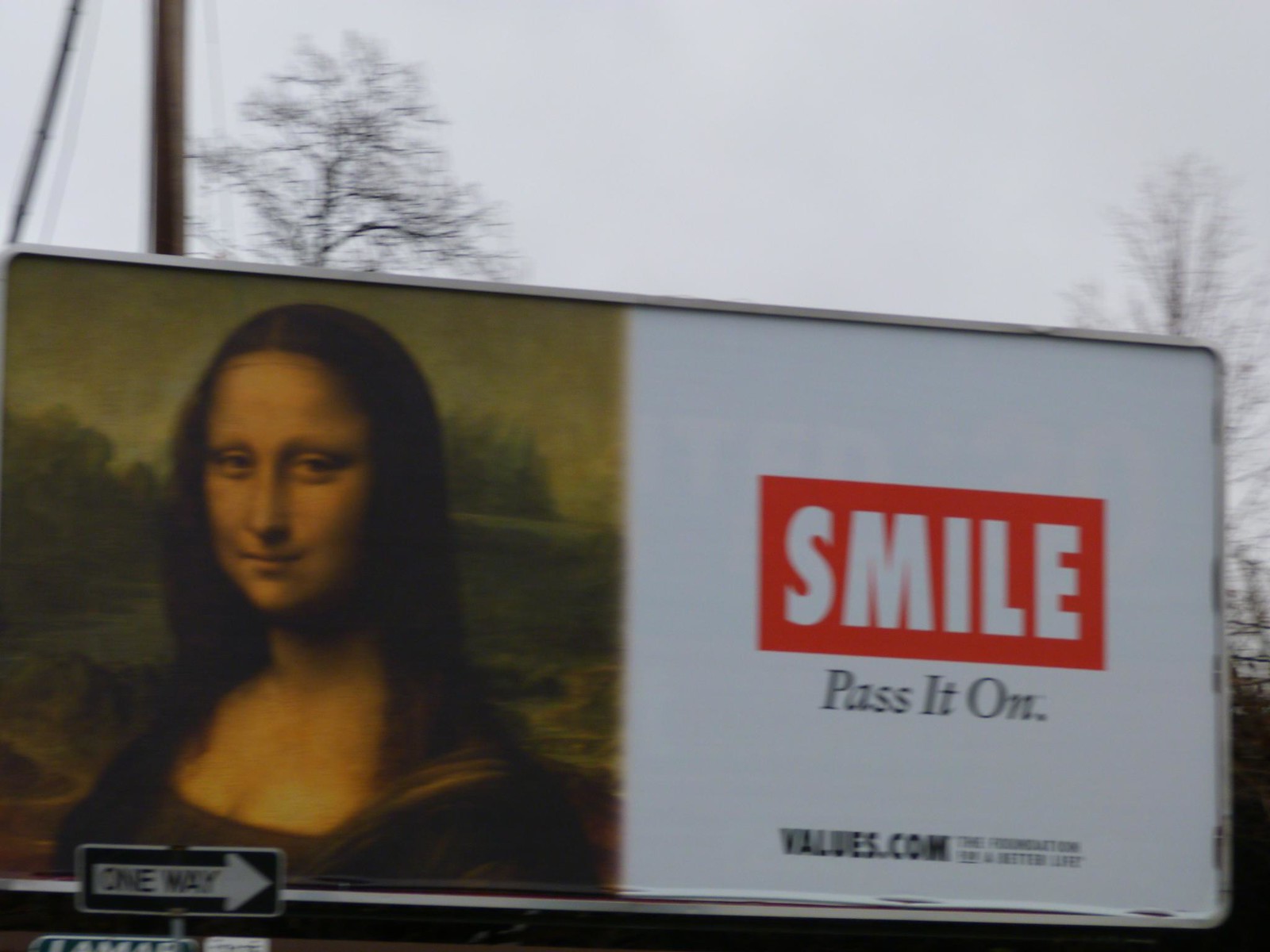The image depicts a rectangular billboard slightly wider than it is tall, occupying the bottom two-thirds of the frame and situated in an outdoor setting during what appears to be late afternoon or early evening, given the hazy gray sky. The billboard is divided into two halves: the left side prominently features the iconic Mona Lisa painting, while the right half has an off-white background with a central red rectangle that bears the word "SMILE" in bold, white capital letters. Below this, smaller black text reads "PASS IT ON," followed by "VALUES.COM" at the bottom, accompanied by some smaller, unreadable text. 

Running vertically about 10% in from the left edge of the image is a telephone pole, from which a wire extends diagonally. Flanking the billboard are barren trees, devoid of leaves, hinting at the winter season. One tree stands to the left behind the billboard alongside the telephone pole, while another occupies the right side of the frame. Additionally, a "ONE WAY" sign with an arrow pointing right is visible at the bottom left of the image.